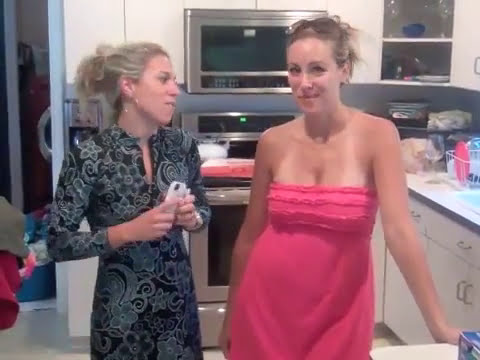In this image, two young women in their early 20s are standing in a well-lit kitchen, possibly taken during a house party. The woman on the right is wearing a strapless pink summer dress, displaying visible bikini tan lines. Resting atop her brown, tied-back hair are a pair of sunglasses, and she is leaning casually against the front counter. The woman on the left is dressed in a black dress adorned with a white floral pattern and has light brown or dark blonde hair pulled back into a ponytail. She holds a smartphone with both hands at chest level, her attention directed towards her friend. The kitchen backdrop features white cabinets and stainless steel appliances, including a microwave over a stovetop and an oven. A dish drainer is visible by the sink, with some utensils in it. The countertops are white, and there appears to be some food on the stove. Through an adjoining doorway, a blue basket filled with laundry is seen, adding a lived-in touch to the scene. One of the women is smirking at the camera, capturing a moment of casual camaraderie.